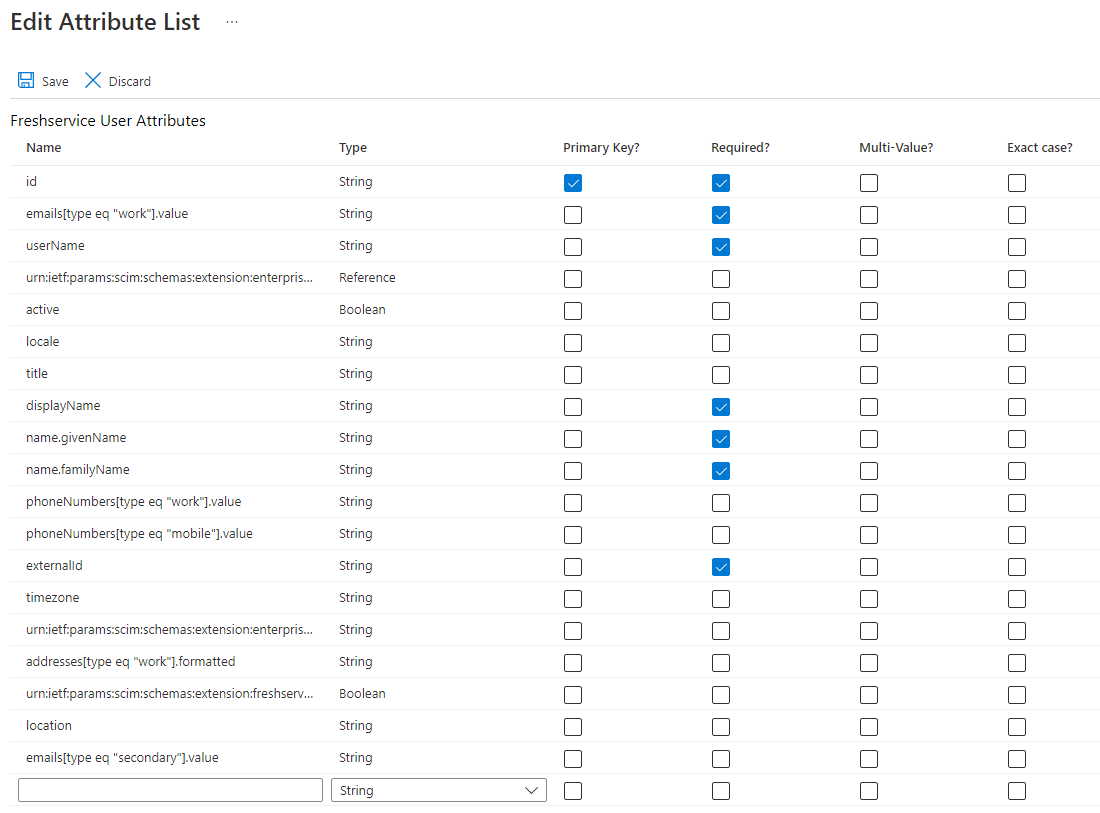The image depicts a detailed user interface, likely from an application dealing with user data attributes. At the top, there are options such as "Edit Attribute List," "Save," and "Discard" with a solid line separating them from the rest of the interface. Below this line, there's a table with six column headers: "Name," "Type," "Primary Key," "Required," "Multi-value," and "Exact Case."

The table is populated with several rows of user attribute data, listed as follows:

1. ID
2. Emails (with sub-attributes: Type=work, Value)
3. Username
4. urnci (with unclear further details)
5. Active
6. Locale
7. Title
8. Display Name
9. name.givenName
10. name.familyName
11. PhoneNumber (with two sub-attributes: Type=work, Value; Type=mobile, Value)
12. External ID
13. TimeZone
14. Address (with sub-attributes: Type=work, Formatted)

The application is identified as "FreshService," and the screen is specifically displaying "User Attributes." The layout and labels indicate a thorough schema for handling user information, emphasizing fields like contact details and localization settings.